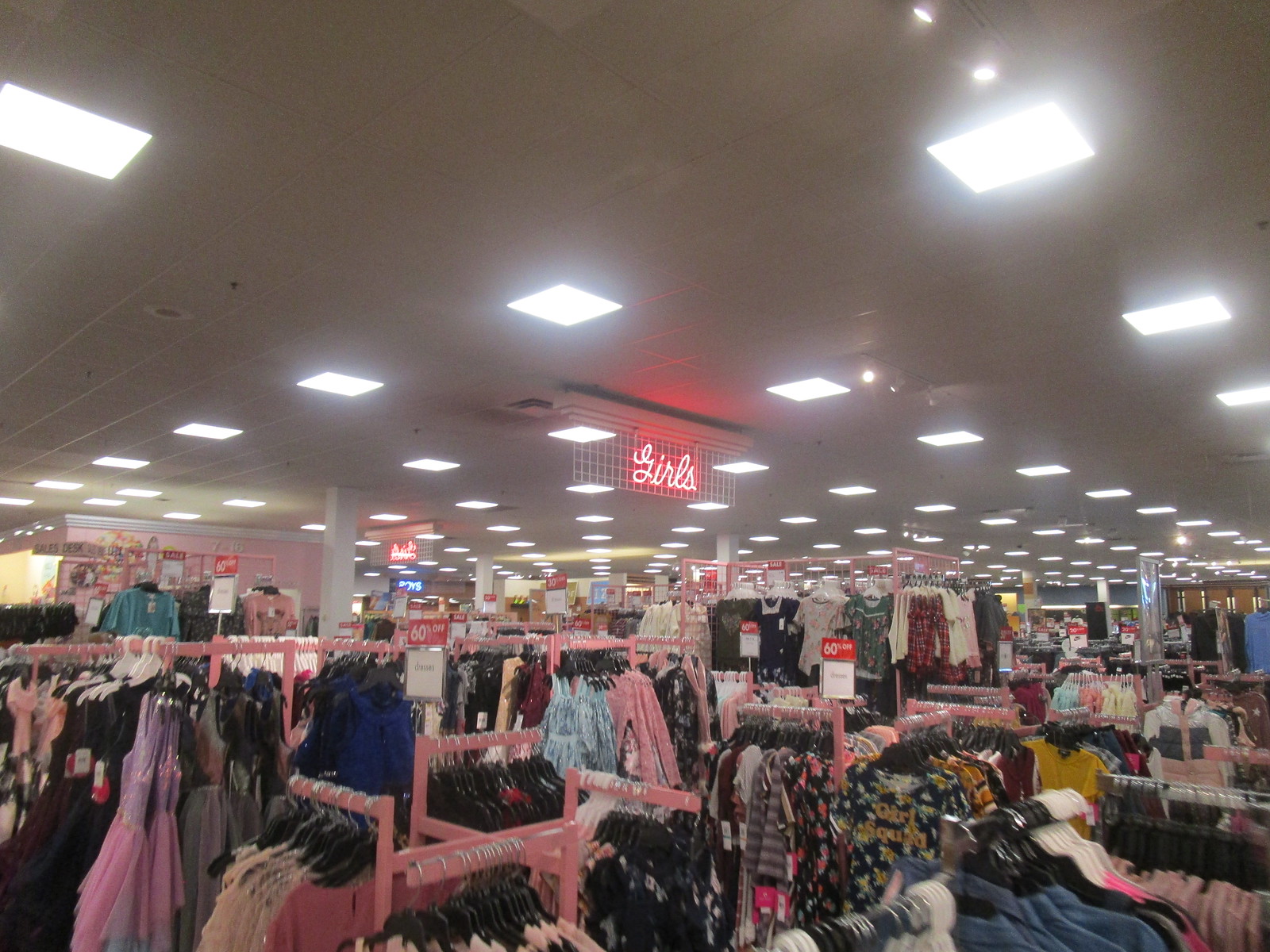The image depicts a wide shot of a large clothing store, possibly a department store, filled with a sea of garments on various racks. The store is brightly lit with numerous ceiling lights, creating a well-illuminated shopping environment. Dominating the top center of the image is an illuminated sign indicating the "Girls" department, featuring white cursive writing on a red background that mimics the style of a neon sign.

In the foreground, a variety of women's clothing is displayed, including multicolored blouses prominently positioned on pink racks with silver hangers. The colors range from beige to blue, adding a vibrant touch to the scene. Dresses are visible at the front of the image, contributing to the diverse selection.

In the background, to the far left, more blouses are arranged on a wall-mounted rack, while additional racks filled with blouses stretch into the distance. Many of the racks are adorned with signs suggesting discounts, possibly indicating "40% off" on select items, inviting customers to take advantage of the deals. Overall, the image captures the bustling, colorful essence of a well-stocked clothing section within a large retail environment.